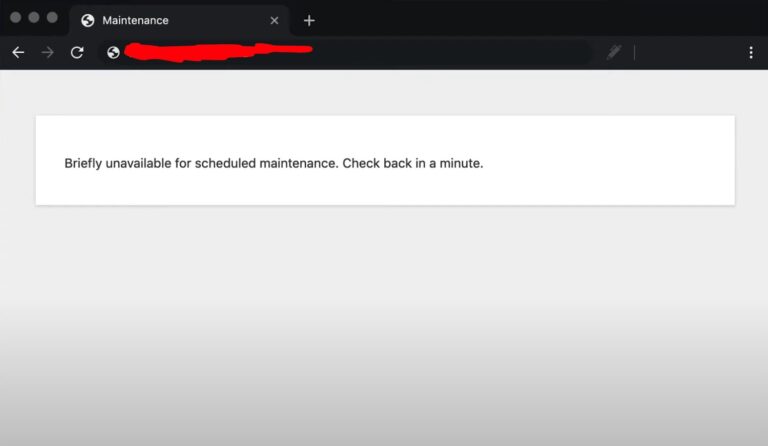The screenshot depicts a web browser with a dark theme active. At the top, the address bar and tab area are completely dark. The visible tab is labeled "Maintenance" in white text, with a small globe icon to its left. Additionally, the top-left corner features three gray dots, while the tab itself includes a gray 'X' and a whitish '+' next to it. The address bar contains a URL that is obscured in red, while on the left side of the address bar, there are back, forward, and refresh arrow icons, all white. To the right of the address bar, there's a gray pen icon followed by three white dots.

The main content of the page is displayed against a gray background that transitions to a darker shade towards the bottom, creating a subtle gradient effect. Centered on this background is a white box containing a message in black text that reads: "Briefly unavailable for scheduled maintenance. Check back in a minute." This concise notification is structured as two sentences within the white box.